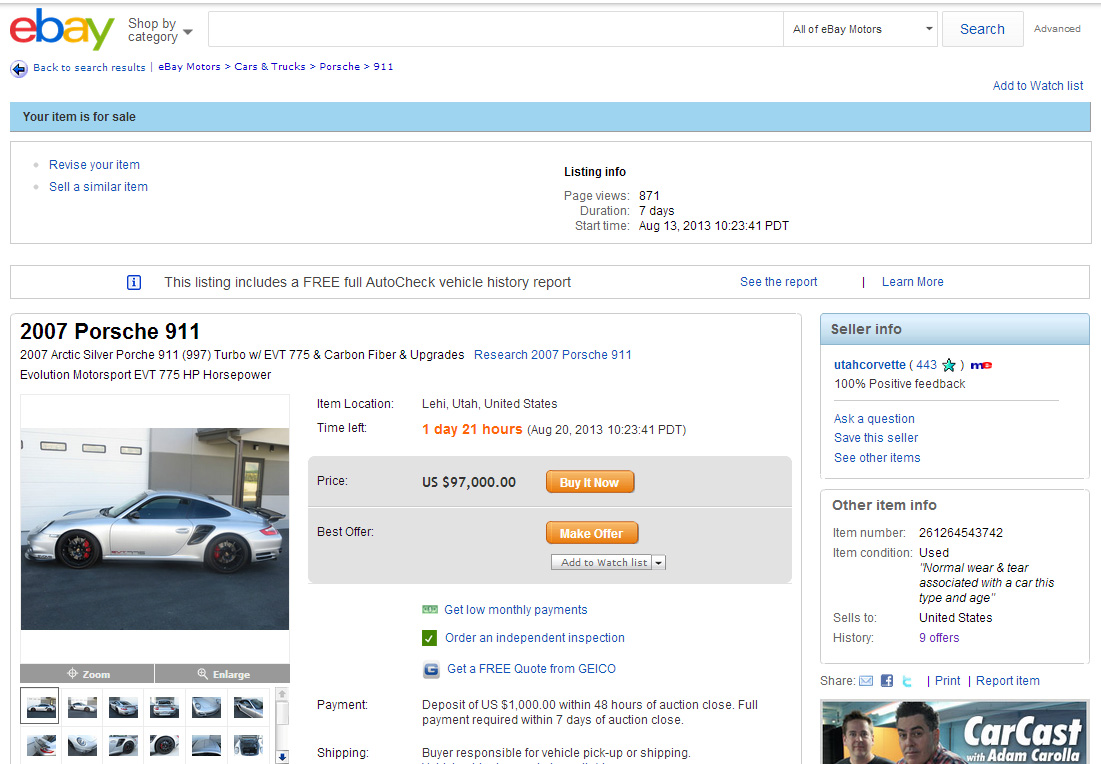An eBay web page is displayed prominently, beginning with the iconic eBay logo at the top left corner. The logo consists of four distinctively colored letters: the "e" in red, the "b" in blue, the "a" in yellow, and the "y" in green. To the right of the logo is a search bar where users can type in their queries.

Beneath the logo, a blue banner spans the width of the page with the message, "Your item is for sale," indicating a seller's perspective. Below this blue banner, within a white box, the listing information is clearly provided.

Dominating the center section of the page is the listing for a 2007 Porsche 911, depicted in a striking silver color. Details about this luxurious car are provided, including its listed price of $97,000. Two actionable buttons are situated beside this: a blue "Buy It Now" button and an alternative option to "Make an Offer," giving potential buyers flexibility in their purchasing approach.

To the far right, the seller's information is prominently displayed. This includes the seller's name, their feedback rating, which boasts a perfect 100% from voters, as well as essential item details such as the item number. Additional information regarding payment and shipping terms is located at the bottom center of the page, providing a comprehensive overview for prospective buyers.